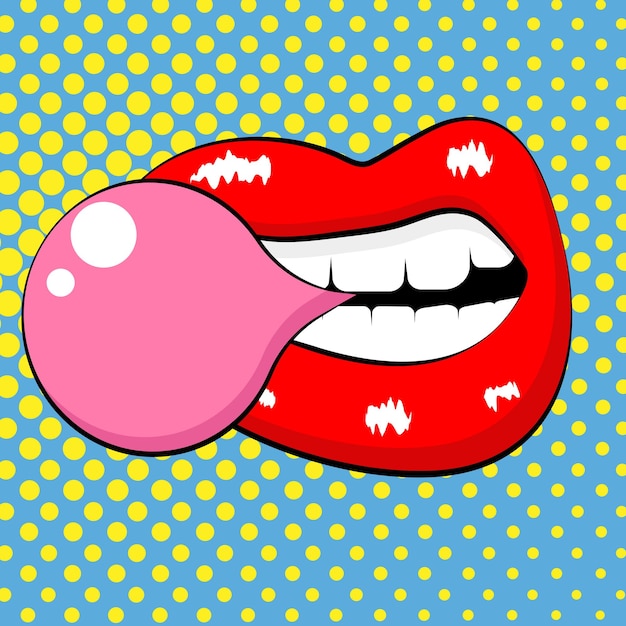This image features a striking, pop art-style graphic reminiscent of a Roy Lichtenstein comic. The central focus is a vivid, oversized set of shiny red lips, reminiscent of the iconic Rolling Stones logo. Unlike the Rolling Stones symbol, these lips are closed, showcasing white teeth while blowing a large, pink bubblegum bubble. Surrounding the lips is a stark black background accented by an array of white squiggly lines, suggesting bits of gum. Encasing this central image is a vibrant blue border adorned with variously sized yellow dots that shift in size—larger on the left side, gradually becoming smaller towards the right. This playful, animated design combines elements of novelty and nostalgia, reminiscent of both vintage candy advertisements and modern emoji graphics.